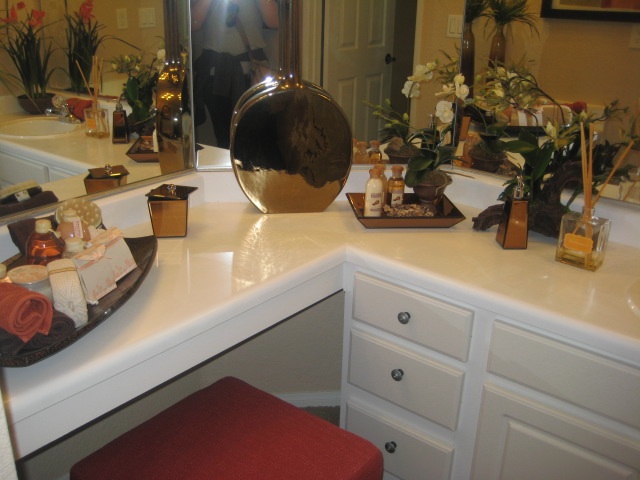A person takes a photo in a well-lit bathroom using a phone or camera, evident from the visible flash glare in the mirror. Positioned on a white vanity that features three drawers, a cupboard, and another drawer, various items are placed neatly. Among these items are an incense holder, some flowers, an orange rolled-up towel, and what appears to be white packages with pink accents, though their exact nature is unclear. Additionally, a small mirror stands in front of the larger mirror on the wall. The vanity is complemented by a red stool that is tucked in, suggesting it is part of the bathroom's setup rather than actively in use.